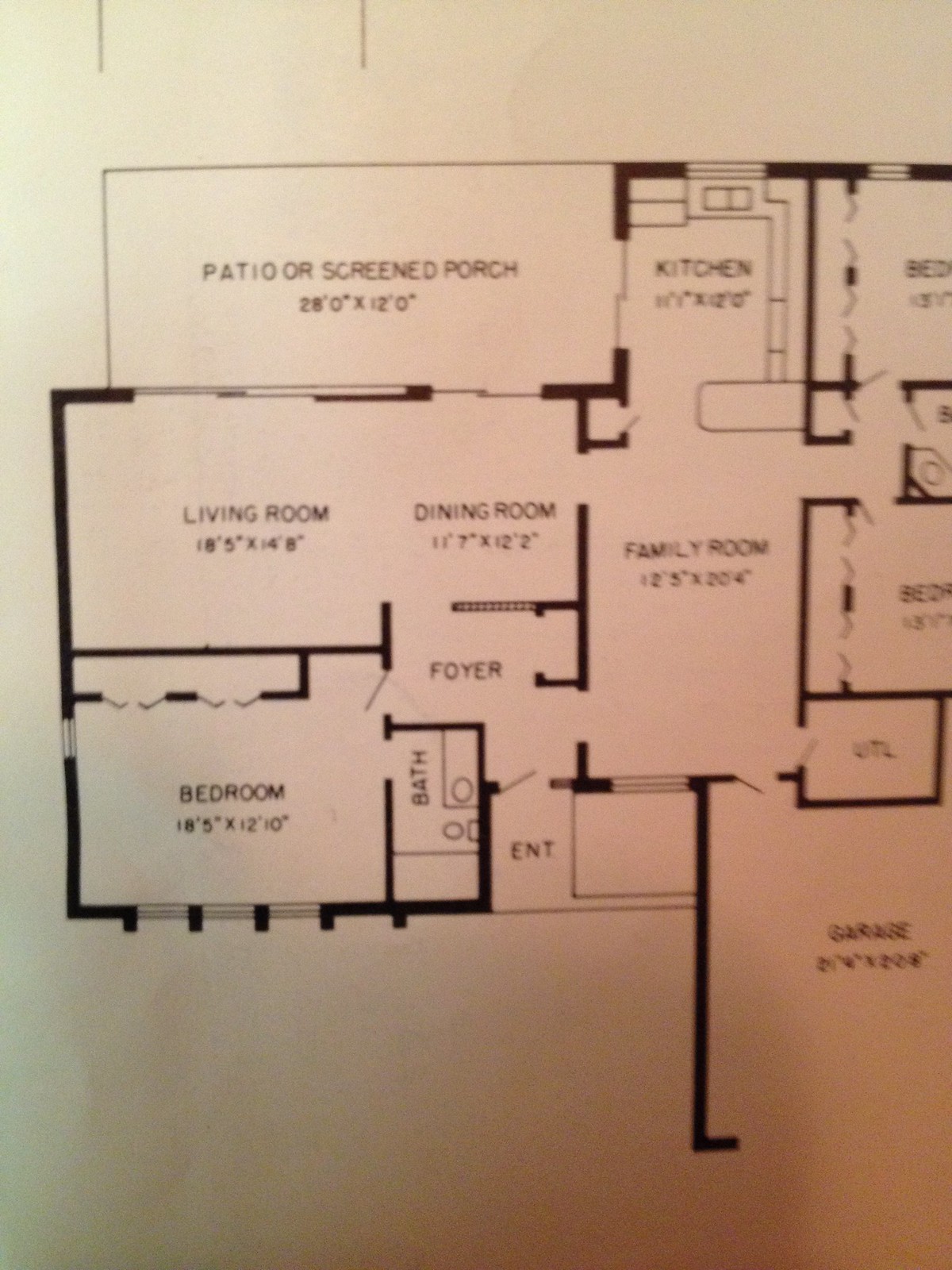A detailed diagram of a residential floor plan is presented in this rectangular image, drawn in black ink on slightly beige, shadowy paper. The layout meticulously shows the dimensions of each room. Starting from the top left corner, there is a patio or screened porch measuring 28 by 12 feet. Directly beneath it is the living room, sized at 18.5 by 14.8 feet, adjoining a dining room. In the lower left corner of the home, there is a bedroom with dimensions of 18.5 by 12 feet, featuring an attached bathroom. To the right of this area, an open family room extends below the kitchen, which measures 11 by 12 feet. The family room itself is 12 by 20 feet. Outlined in the lower right corner is the garage, although its dimensions are not legible. Additionally, two more bedrooms are indicated on the right side of the image, one positioned above the other, along with a small utility closet labeled "UTL." The lower right-hand corner of the image is obscured by a golden brown shadow, adding to the overall unclear quality of the diagram.